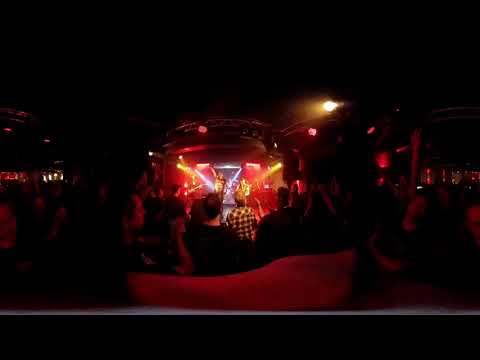The image is a smaller-sized square photograph set within a mostly black background at the top and bottom. Taken from a first-person perspective in a dark indoor setting, possibly a music auditorium or bar, it captures the scene of what appears to be a concert. The stage, positioned at the center in the distance, is illuminated by vibrant stage lights in shades of red, blue, and gold, along with a white spotlight shining from above. The band on stage is difficult to see clearly due to the distance and lighting, making their features indistinguishable. In the foreground, the backs of people's heads make up the audience, all seated and facing the performers. The atmosphere is filled with the presence of girders or rafters around the stage, enhancing the structural ambiance of the venue. The overall color palette includes black, brown, beige, tan, red, blue, yellow, and white, contributing to the dynamic yet dimly lit concert scene.